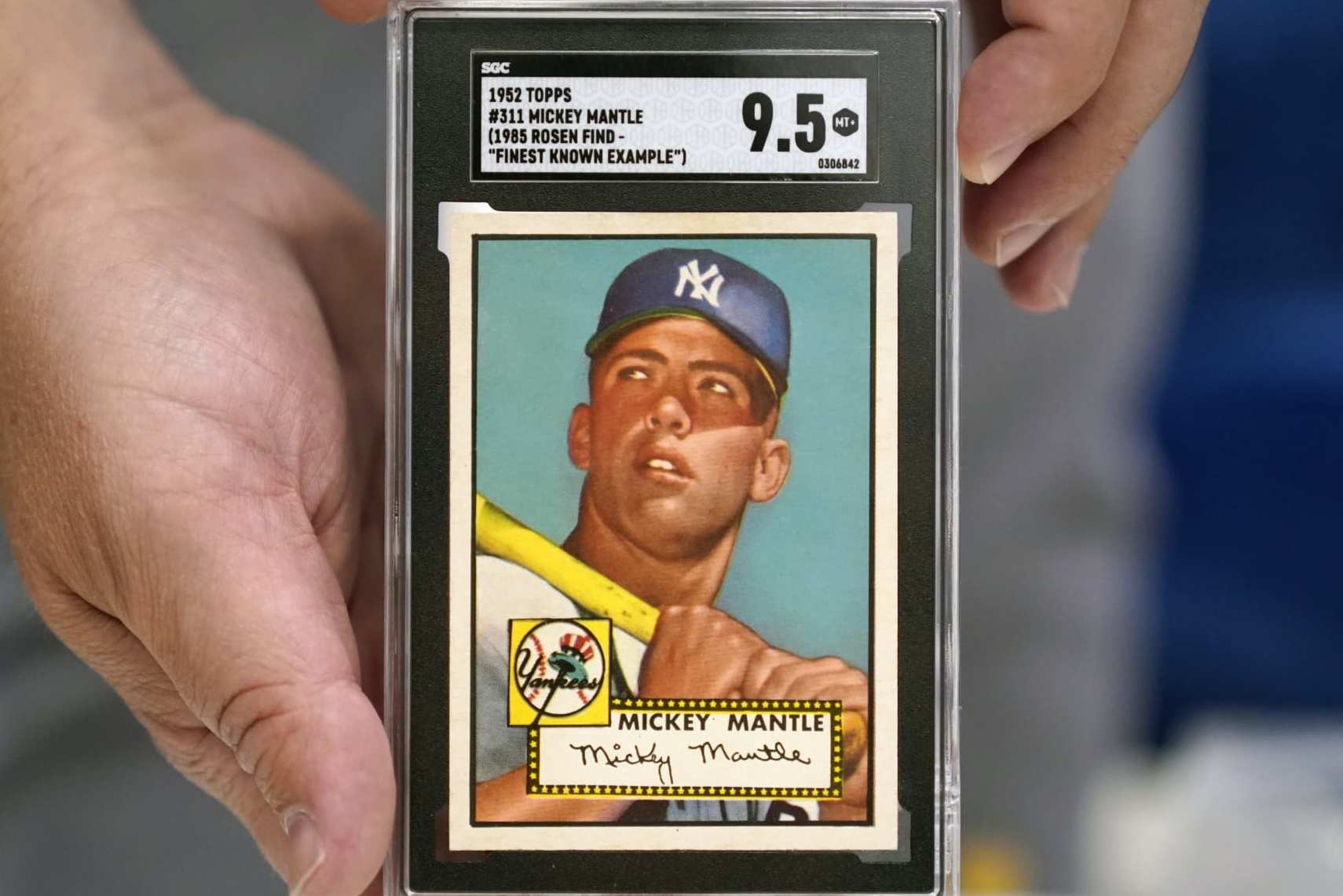In this detailed image, we see a rare and valuable baseball card encased in a clear protective case, being held by someone's hand. The card is a 1952 Topps #311 Mickey Mantle, highly graded at 9.5, making it one of the finest known examples. The legendary player Mickey Mantle is depicted on the card, wearing a New York Yankees blue cap with white lettering, and holding a yellow bat over his right shoulder. The card's title, "Mickey Mantle," is prominently displayed alongside a black box with yellow stars and his authentic signature. The background is blurry, ensuring all focus remains on this rare and expertly preserved piece of sports memorabilia.